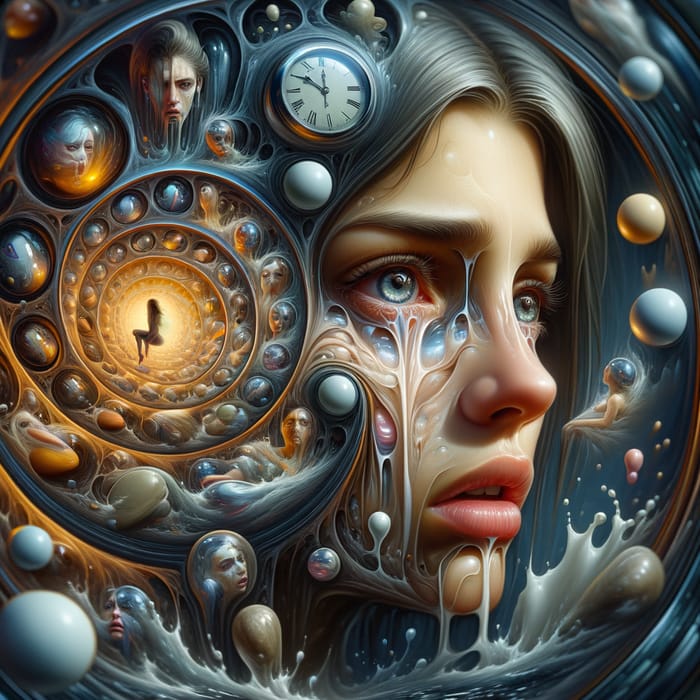The image is a detailed digital artwork featuring a central abstract depiction of a female face. The woman's face, predominantly pale with a melting appearance, is surrounded by intricate elements that merge realism with surrealism. Her blue eyes and pointy nose are defined, while her hair takes the form of a swirling, spiral shell. This shell is dotted with multiple circles, each containing miniature melting faces identical to hers. Centered within the shell, a woman is seated, bathed in the glow of a radiant yellow circle, indicating a clock set at 12:50. The woman's grayish-brown or silver-gray hair flows downward, blending into light blue and caramel cream-colored rivulets that resemble tears. These tears transition into a surrounding watery vortex, interspersed with floating faces and cubic 3D balls. Additional faces appear within splatters of liquid at the bottom of the frame, as if the tears have turned into a splashing river. The predominant colors—silver, gray, blue, and hints of orange—add to the ethereal and mesmerizing quality of the artwork.